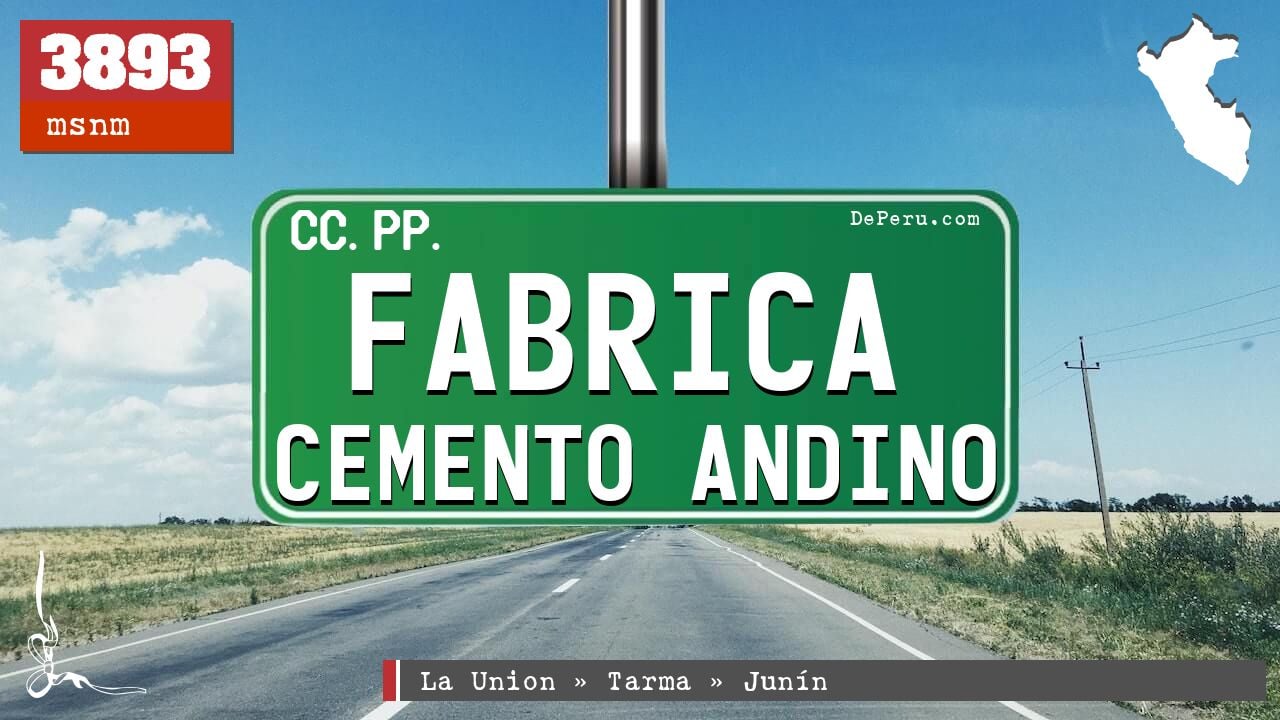The image is an advertisement or graphic related to travel, seemingly in Peru. The main visual element is a green rectangular road sign with rounded edges, hanging from a shiny metal pole. The sign displays white text that reads "cc.pp" at the top and "Fabrica Cemento Andino" in larger letters. The top right corner of the image features a white graphic of Peru, and the website "deperu.com" is visible, reinforcing the Peruvian context. In the top left corner, a red box with white text displays "3893 MSNM". The background showcases a flat highway bordered by sparse plains with minimal green vegetation and no significant trees, all under a blue sky with some white clouds. At the bottom, a gray bar with a red and white line on the left displays white text reading "La Union" followed by arrows pointing to the right with "Tarma" and "Junin" also indicated with arrows. There is a secondary pole with wires on the right side of the road. This detailed representation suggests a rural setting with an emphasis on travel routes or directions in Peru.